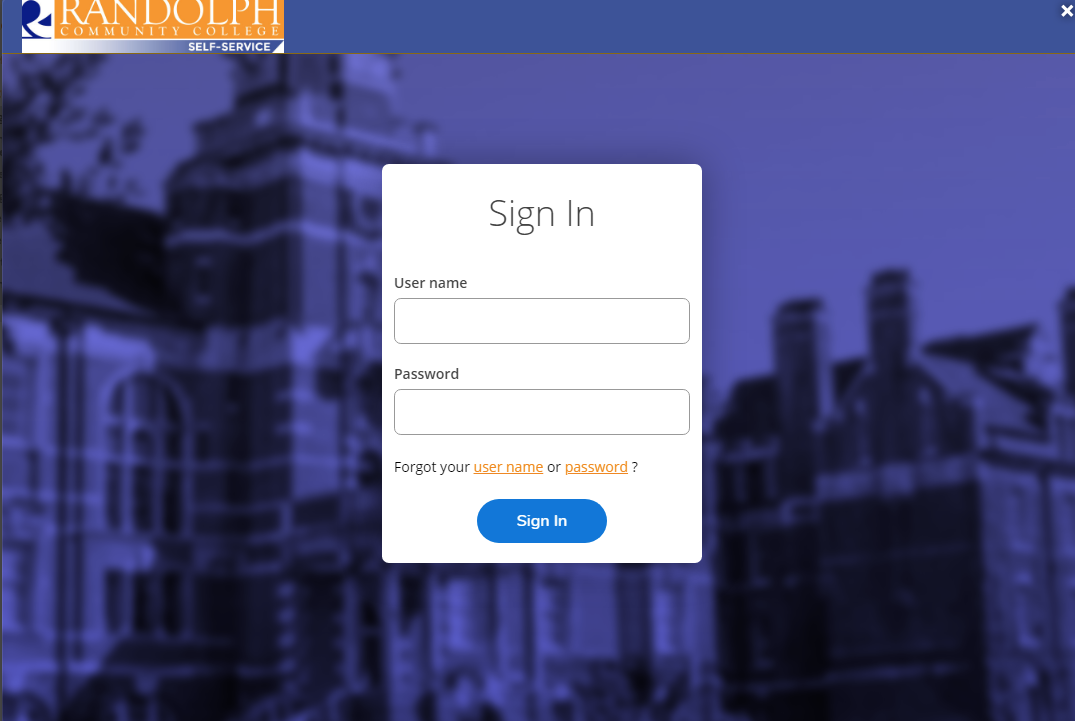The website page features a blue background with a slightly blurred image of a college campus, displaying at least two buildings. In the top-left corner, there is an orange banner with "RANDOLPH" written in capital letters. Below this, within the same orange banner, "Community College" is also displayed. Directly underneath, a white banner transitions to blue on the right side, where "SELF SERVICE" is prominently written in white capital letters.

In the center of the page, a white pop-up box is displayed. The top center of the pop-up contains the text "Sign In" in black letters. Below this, there are fields to enter a username and a password. Additionally, if a user forgets their username or password, there is a clickable link within the pop-up for assistance. After entering the required information, users can click "Sign In" to proceed.